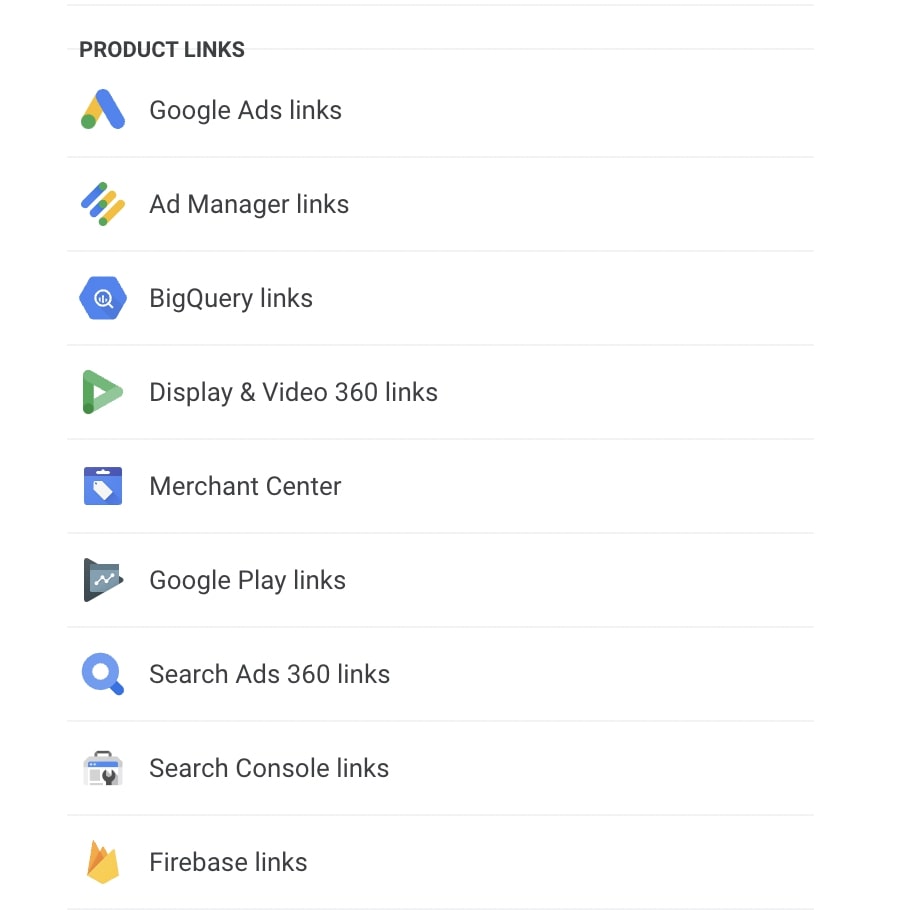This detailed image showcases a list of Google product links laid out vertically. At the top left, the title "Product Links" is prominently displayed in bold black letters. Extending from the 'S' in "Product Links" to the right edge of the page is a thin grey line.

1. **Google Ads Links**: This appears first in the list with an accompanying icon resembling an upside-down "V". The icon features a blue section on the right side and a smaller blue circular tip at the lower end on the left.
   
2. **Ad Manager Links**: Following, this entry has an icon composed of three lines in alternating blue and yellow hues, tilted at approximately 70 degrees.

3. **BigQuery Links**: This link is denoted by a blue octagon with a stylized magnifying glass set in the center.

4. **Display & Video 360 Links**: This is represented by a right-facing green triangle icon.

5. **Merchant Center**: Next, this link's icon is a blue square with a white price tag positioned in the middle.

6. **Google Play Links**: Recognizable by its icon, the classic play button pointing to the right.

7. **Search Ads 360 Links**: Featuring a thick blue magnifying glass icon.

8. **Search Console Links**: This link is symbolized by an icon that resembles a briefcase.

9. **Firebase Links**: Concluding the list, this displays an icon with triangles arranged to depict flames.

Each product link is distinguished by unique icons and a structured vertical alignment, making the entire ensemble visually organized and easy to navigate.